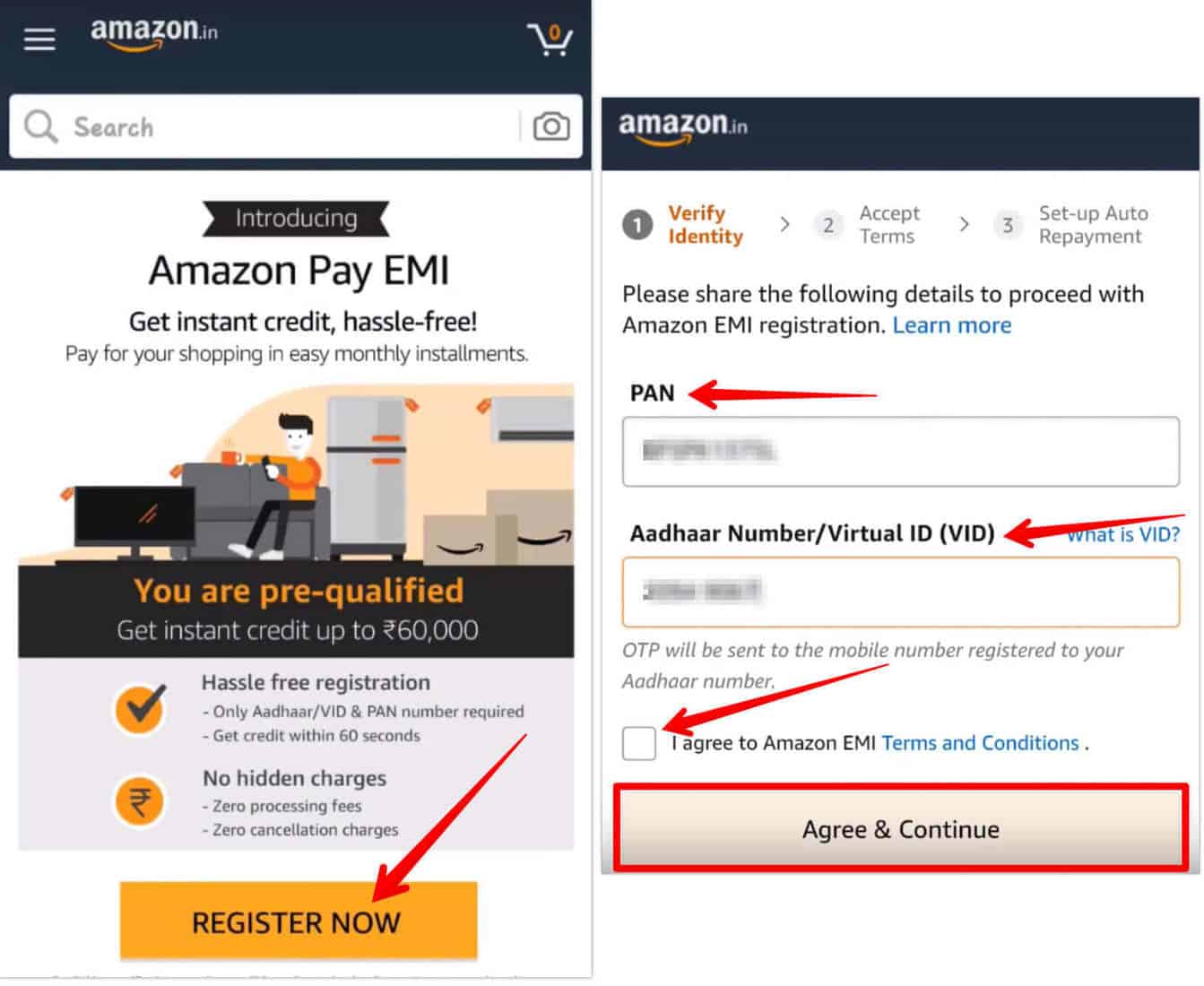### Detailed Caption:

The image seems to be a step-by-step instructional guide found on a website like Amazon, designed to explain the process of registering for Amazon Pay EMI. 

**Left Panel:**
1. **Header:**
   - In the top left-hand corner, it features the "Amazon" logo with the hamburger menu icon (three horizontal lines). 
   - To the right-hand corner, there's a cart symbol showing "0" items.
2. **Content:**
   - The top part of the panel introduces "Amazon Pay EMI." It states, "Get instant credit, hassle-free, pay for your shopping in easy monthly installments," and highlights that "You are pre-qualified" written in orange text.
   - Below this, there's an illustration of a person shopping or looking at their phone, with Amazon boxes beside them.
   - Additional details include:
     - "Get instant credit up to €60,000" (assuming the Euro symbol is used here).
     - "Hassle-free registration" represented by an orange circle with a blue checkmark.
     - Specifications: "Only Aadhaar/VID and PAN number required, get credit within 60 seconds."
     - Benefits: "No hidden charges, zero processing fees, zero cancellation fees."
   - At the bottom, a prominently featured orange button with a red arrow pointing to it says "Register Now."

**Right Panel:**
1. **Header:**
   - In the top left-hand corner, the "Amazon" logo is present.
2. **Steps:**
   - The panel is divided into three numbered steps in gray text:
     1. **Verify Identity:** This appears to be the current step.
     2. **Accept Terms**
     3. **Set Up Auto Payment**
3. **Details for Verification:**
   - Instruction to "Please share the following details to proceed with Amazon EMI registration."
   - "Learn More" for additional information.
   - Fields for entering details:
     - **PAN:** With a red arrow pointing to a text box for user input.
     - **Aadhaar number/Virtual ID (VID):** Accompanied by an explanatory link, "What is VID?" and a text box for input.
   - It also mentions that an OTP will be sent to the mobile number registered with the Aadhaar account.
   - A checkbox, indicated by a red arrow, that needs to be ticked, labeled "I agree to Amazon EMI terms and conditions."
4. **Final Step:**
   - A red-outlined box at the bottom states "Agree and Continue," which presumably initiates the next step in the process.

This thorough instructional image aims to guide users clearly through registering for Amazon Pay EMI, ensuring they understand each step and the requirements needed.